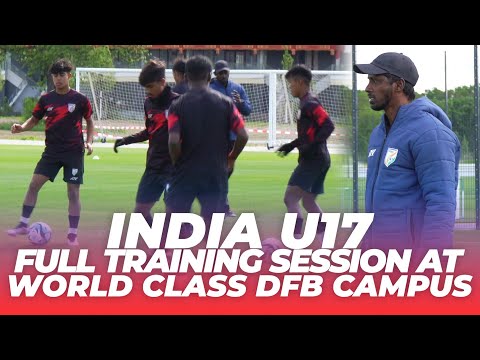The image appears to be a screengrab from a video or a thumbnail, capturing a vibrant scene on a green soccer field with a backdrop of green trees and a white goalpost. Dominating the bottom of the image is bold white text that reads "India U-17 full training session at world-class DFB campus." This text is set against a red background that gradually fades from solid red to transparent as it progresses upwards. The photo features a composite of two scenes blended together: on the left, a cluster of soccer players in black and red uniforms engaged in practice, with a blue-clad coach standing in the background; on the right, a side profile of the same coach, identifiable by his blue jacket and dark baseball cap, gazing to the left. The players are gathered around a soccer ball on the lush grass with a distant athletic building visible behind the net, emphasizing the organized and professional nature of the training session.